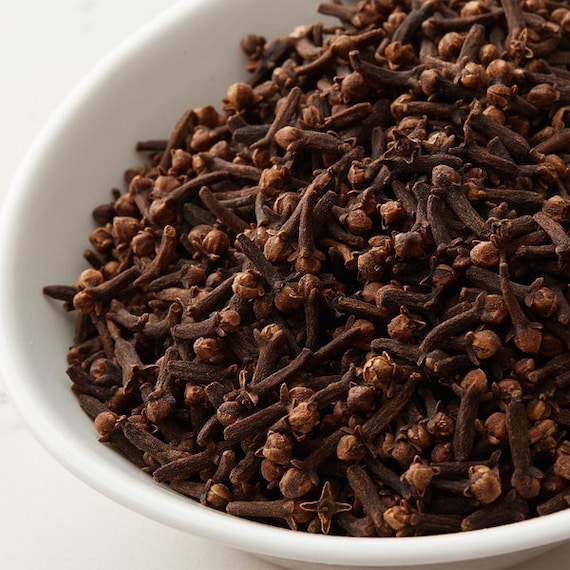This close-up photograph captures a white porcelain bowl filled to the brim with dried cloves, sitting on a white background, likely a table or countertop. The image is zoomed in so closely that a significant portion of the bowl is cut off, particularly along the top right and right-hand sides. The cloves are in various sizes and shapes, resembling small brown twigs with smooth, thin stems and bulbous, bumpy heads. Each of the cloves has a distinct structure, featuring a prominent bulbous top with four spikes around it. The spices are densely packed, with hundreds of them tilting over the bowl's edge. The detailed focus on the cloves reveals their intricate textures and makes the spices visually intriguing, suggesting a tactile quality that invites you to imagine the sensation of running your fingers through them.